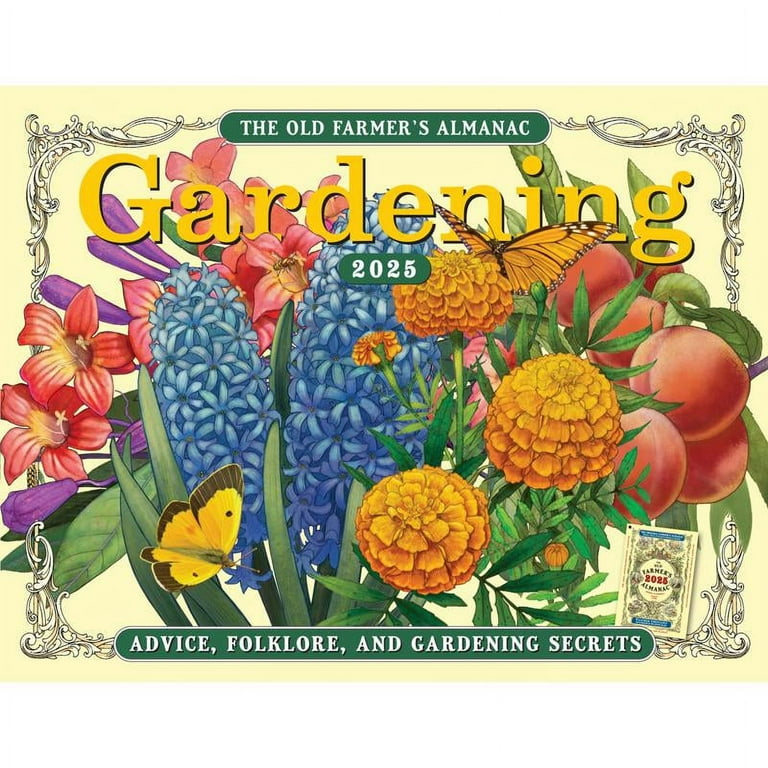This detailed poster for "The Old Farmer's Almanac: Gardening 2025, Advice, Folklore, and Gardening Secrets" features a beautifully vibrant and inviting scene. At the top and bottom of the poster, "The Old Farmer's Almanac" is prominently displayed in a green marquee style. The word "Gardening" is highlighted in large yellow font at the top, with "2025" beneath it in a green circle. The text "Advice, Folklore, and Gardening Secrets" is similarly placed in a green circle at the bottom.

The central image bursts with color, showcasing a rich variety of flowers and fruits. A striking collection of marigolds, hyacinths, and other red, blue, purple, pink, and orange flowers bloom amidst lush green foliage. The scene is further enlivened by the presence of fruits, including branch-hanging peaches and clusters that resemble tomatoes. Adding to the charm, two butterflies—a yellow one with black tips and an orange monarch—dance around the blooms.

The entire scene is set against a pale yellow background with an ornate white border reminiscent of a vintage diploma. In the bottom right corner, a small picture of "The Old Farmer's Almanac" adds a touch of authenticity and tradition to this picturesque advertisement for the 2025 gardening edition.